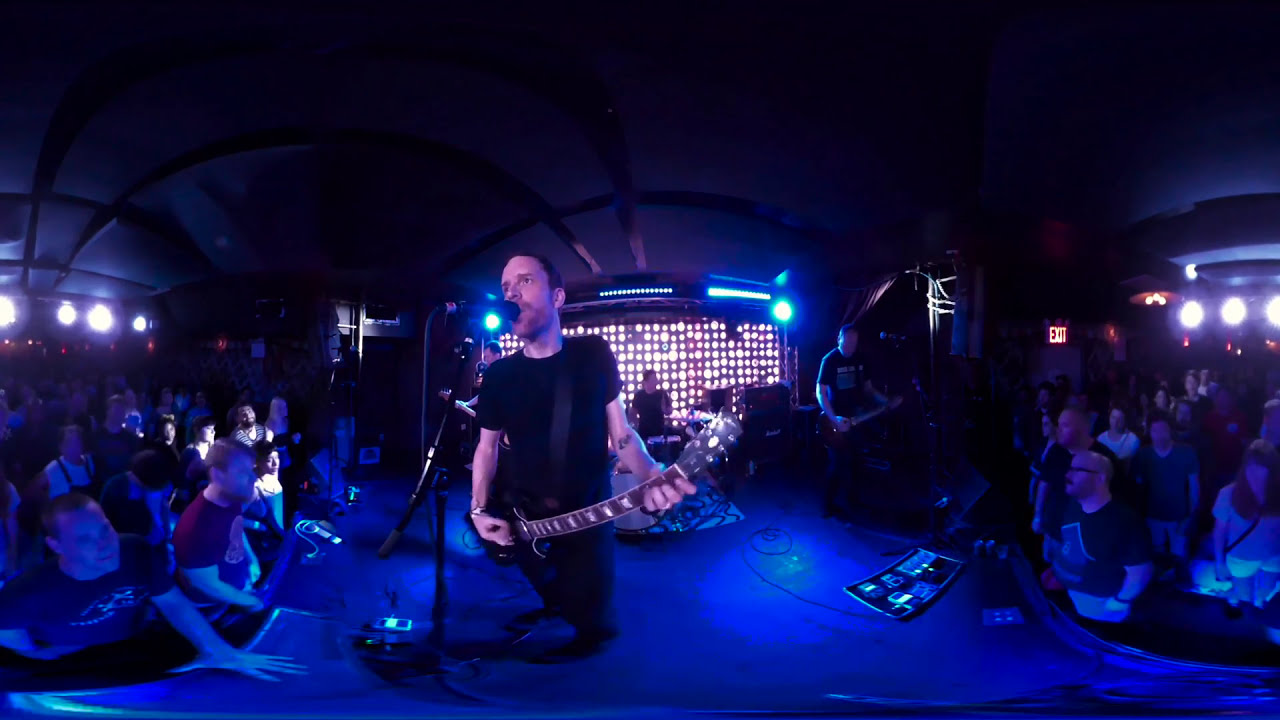The photograph captures an indoor concert, possibly in a nightclub or music venue. The scene is dimly lit, predominantly with blue lighting, creating a moody atmosphere. At the forefront, left of center, stands a white male singer dressed in a black t-shirt, black jeans, and black shoes. He holds an electric guitar and is engaged with the microphone, peering into the crowd on his left. Behind him, a drummer, identifiable by tattoos on his left arm and a watch-like accessory on his right wrist, is partially visible. To the right of the stage, another musician, possibly a bassist, also dressed in black, contributes to the performance. The audience surrounds the stage on both sides, primarily consisting of white men in their 20s and 30s, with some women dispersed among them. The overall color scheme of the image is dominated by shades of blue, white, and black, indicating a carefully controlled lighting design typical of live music events.